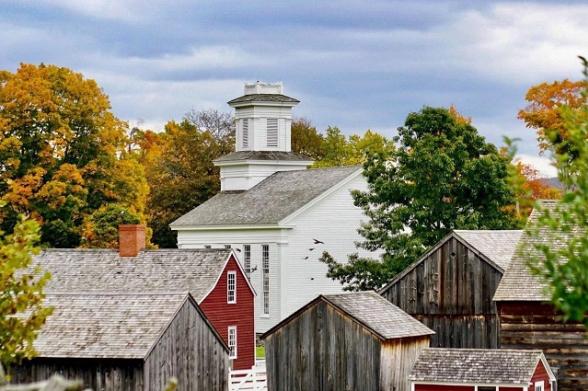The image captures a picturesque scene featuring an old-fashioned, historical property with a variety of structures. Dominating the center is a large white building with long windows along its side and a distinct white chimney structure protruding from its grey roof. In the foreground, there are five small buildings, which resemble sheds or shacks, constructed from dark brown and dark greyish wood, with paneling visible. To the right of the white building stands a smaller red shed, while off to the left, there is a larger red house-like structure. Scattered among these buildings are trees with mostly green leaves, though some are beginning to turn orange, signaling the change of seasons. The sky overhead is a vibrant blue with patches of white clouds drifting, casting a slightly dark hue over the scene. This charming tableau is surrounded by lush greenery, evoking a serene and timeless ambiance.